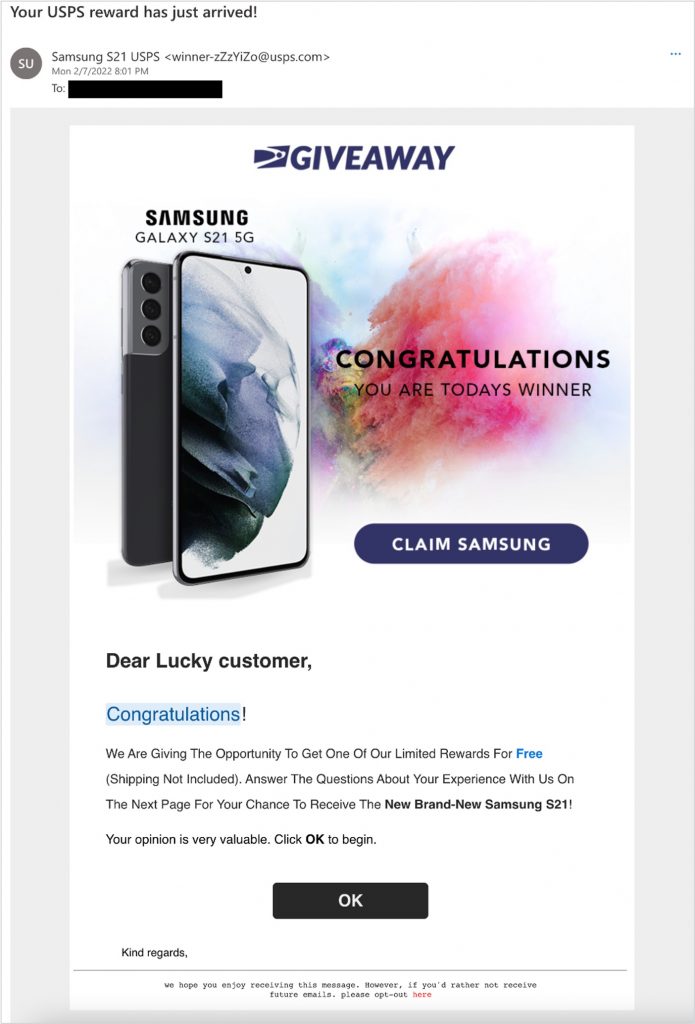Caption: 

A suspicious email, purportedly from USPS but likely a phishing attempt, claims the recipient has won a Samsung Galaxy S21 5G. The email, sent by "SamsungS21UPS" on Monday, February 27, 2022, at 8:01 PM, features a USPS logo and the heading "Giveaway" at the top. It congratulates the recipient, declaring them "today's winner," and includes a button labeled "Claim Samsung." The email further instructs the recipient to answer some questions about their experience with the sender for a chance to receive the Samsung S21, emphasizing that shipping is not included. A concluding note says "Kind regards," but the message raises suspicion due to inconsistencies, such as the email supposedly being from USPS while offering a prize from Samsung, suggesting it might redirect to a phishing site to steal personal information.